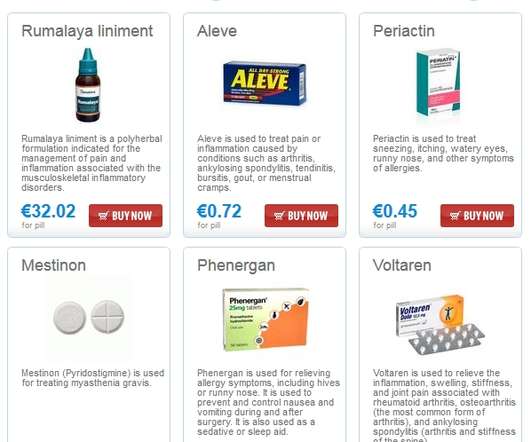Below is a detailed and cleaned-up caption for the described image:

---

The website showcases a grid of six advertisement boxes, each outlined in gray against a white background. 

1. **Rumalala Liniment:** The first box, in blue with yellow lettering, depicts a small bottle with a high-top screw-off cap. Priced at 32.02 units (currency unspecified), this liniment also features a "Buy Now" button in red.

2. **Paracetam:** The second box displays a white and blue box of medication. Similar to the first, it is priced in light blue text (non-USD) and includes a "Buy Now" button in red.

3. **Mastinon:** The third box contains an image of pills, shown from both the front and back. It follows the same pricing method and includes a "Buy Now" button in red.

4. **Phenogan:** The fourth box presents an orange, green, and white packaging of the medication, accompanied by a description of its use.

5. **Mastinon:** The fifth box repeats the Mastinon medication description and imagery of the front and back of the pills.

6. **Voltaren:** The final box features a white and orange packaging of Voltaren, showing the pills in their tray. Like the others, it includes a detailed description beneath the image.

Each box includes a short description of the medication it advertises, providing consumers with essential information at a glance.

---

This detailed caption ensures clarity and thoroughness, giving an accurate representation of the image described.